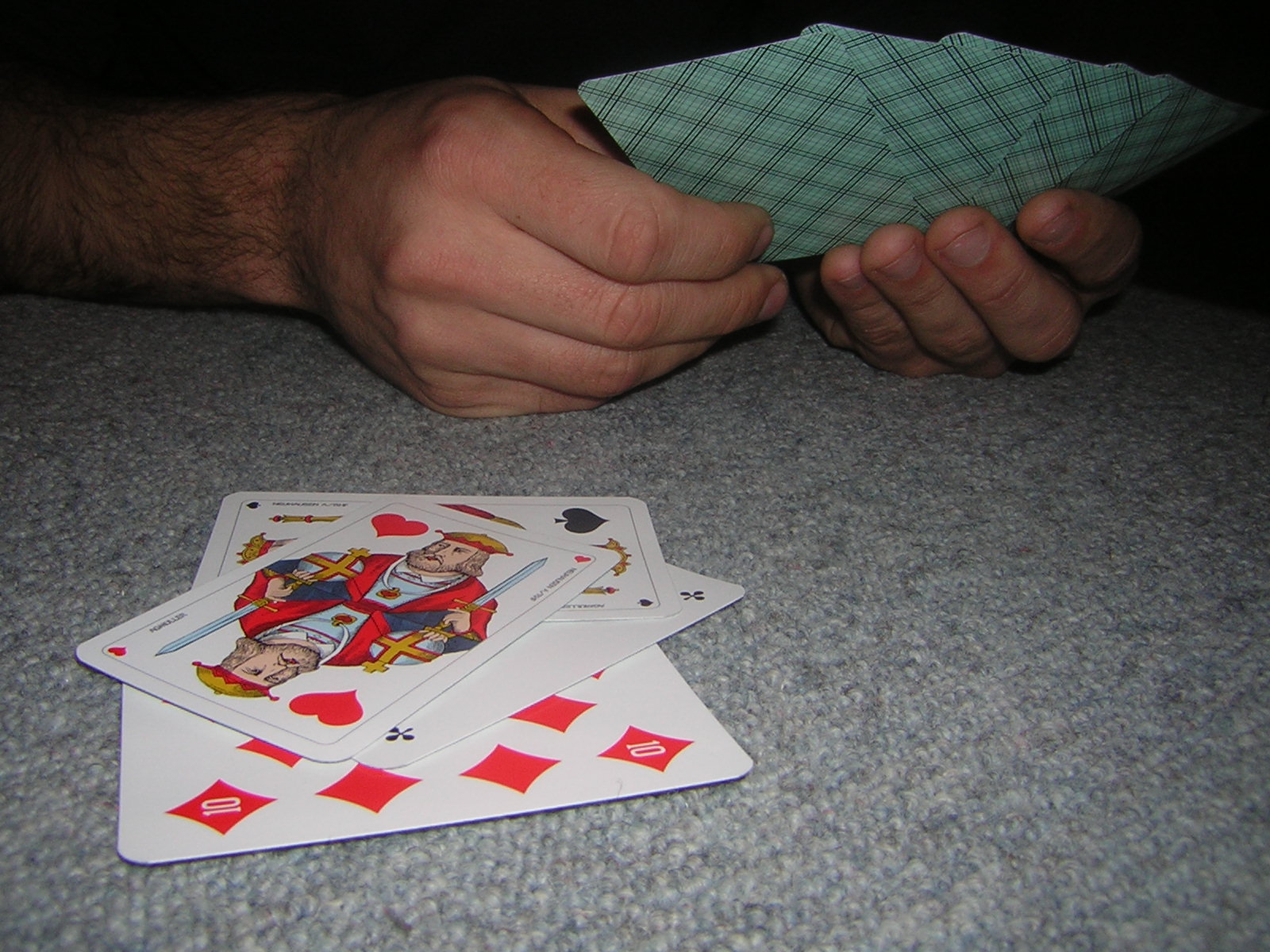A photo captures an intense moment during a card game, likely a solo session of solitaire, spread out on a gray carpeted floor. The image focuses on a pair of hands, revealing the player to be a white individual, holding four or five cards with green backs. The face-up stack of cards in play displays a king of hearts on top, followed by a black heart card, an unknown club card, and a ten of diamonds at the bottom. The obscured ranks of some cards add a layer of mystery to the scene, while the visible cards hint at the strategic decisions being made by the player.